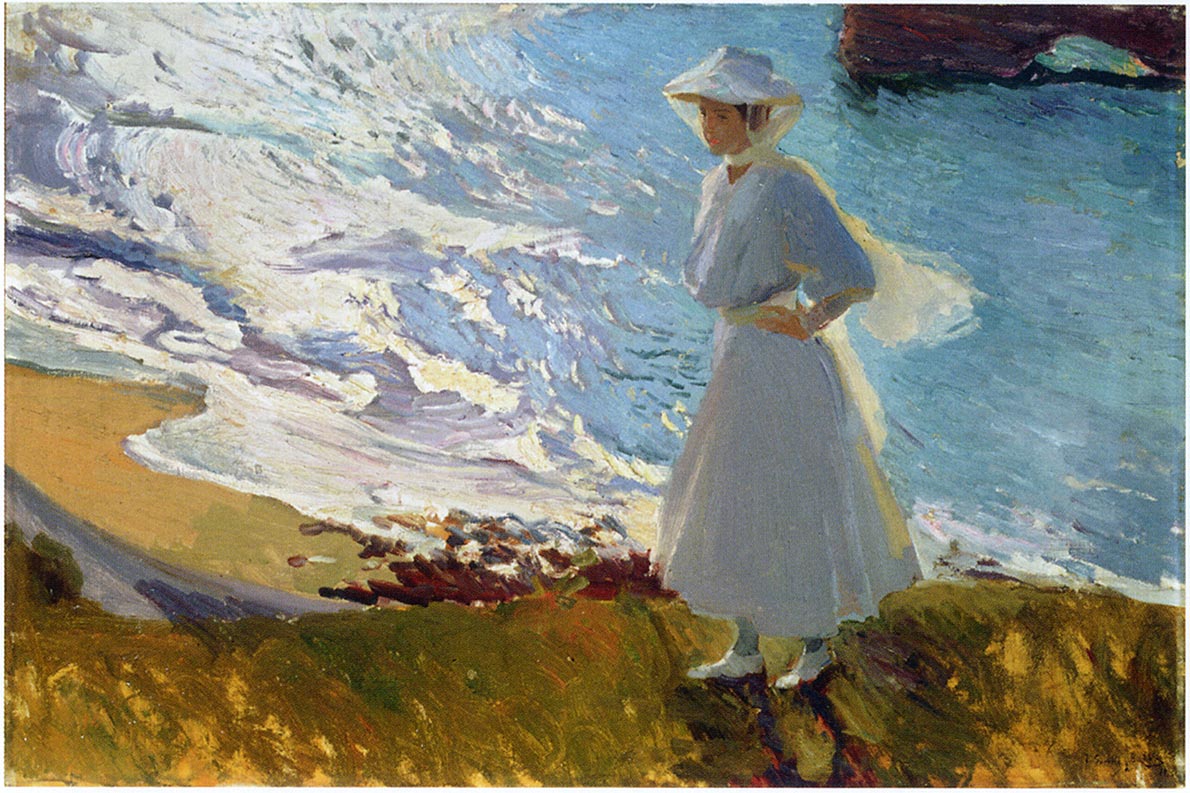This detailed painting depicts a woman dressed in a full, flowing white summer dress, complemented by a white hat with a scarf that elegantly flows over her back. She stands on a green hill tinged with shades of yellow and dotted with some brown plants, indicative of the grass or weeds native to the area. The woman’s white shoes peek out beneath her long skirt, which nearly reaches her ankles. Her gaze is directed to the left side of the painting, conveying a sense of contemplation or observation.

In the background, beyond the hill, a serene beach scene unfolds. The water near the shore is painted in predominantly blue tones, with light reflecting off the gentle waves and creating patches of white where the waves meet the shore. The sandy beach is a mix of gray tones, adding depth to the foreground water. Notably, in the upper right-hand corner of the painting, a remarkable rock formation with a hollow section at its base emerges from the water, adding an element of intrigue. This masterfully executed piece allows viewers to appreciate the texture of the artist's brush strokes, bringing the scene vividly to life, reminiscent of a Victorian-era seaside moment.